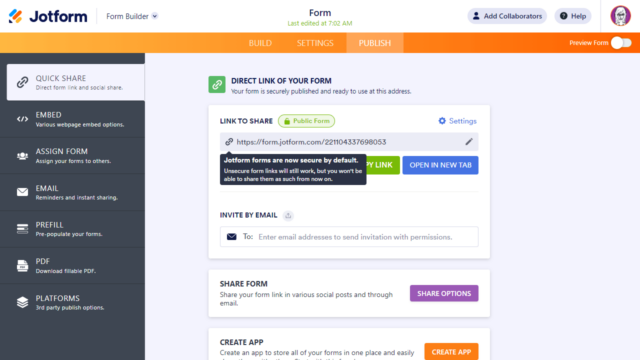This is a detailed screenshot of someone using JotForm, a form builder application, taken at 7:02 a.m. At the very top white navbar, from left to right, are icons for "Add Collaborators," "Help," and a user profile icon. Below this is a horizontal header bar with an orange gradient that lightens towards the left and darkens towards the right. This bar features options labeled "Build," "Settings," and "Publish," with the "Publish" section highlighted by a lighter shade of yellow. To the far right, there is a toggle switch labeled "Preview Form," which is currently turned off.

On the left side of the screen, there's a vertical menu bar with the "Quick Share" option highlighted. Under this section, there are icons representing different sharing functions: a chain link icon for "Embed," which shows left caret, right caret, and slash symbols; "Assign Form" with an envelope icon; "Pre-Fill" with bar graph icons; "PDF" with a printer icon; and "Platform" with three stacked papers icon for third-party publishing options.

The main area to the right displays the "Quick Share" section. Here, a green square contains the text "Direct link to your form" indicating that the form is securely published and ready to use at the provided URL: form.jotform.com/221104337698053. There is a lock icon on the "Link to share public form" button, which is followed by a "Settings" button and a speech bubble stating, "JotForm forms are now secured by default. Unsecured form links will still work, but you won't be able to share them as much from now on." Below this message, an obscured green button likely saying "Copy Link" and a visible blue button that reads "Open in New Tab" are present.

Further down, there is an "Invite by Email" section where users can enter email addresses to send invitations with permissions. A floating field beneath this for "Share Form" allows sharing the form link via various social channels and email, indicated by a purple button labeled "Share Options." At the bottom of the image, partially cut off, is a section suggesting the creation of an app to store all forms in one place with an orange button labeled "Create App."